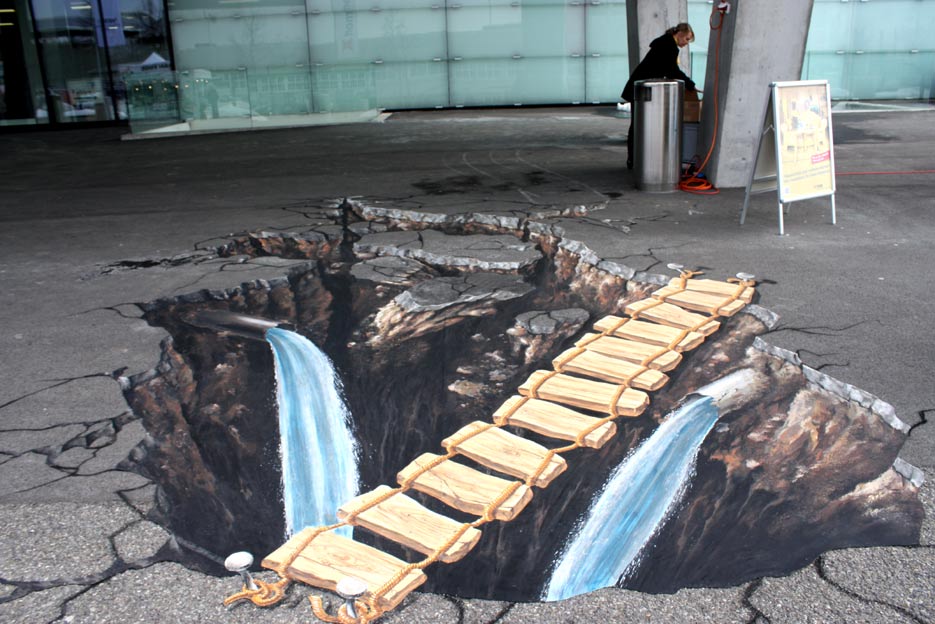The photograph showcases a striking piece of street art painted on an outdoor, urban concrete surface that convincingly mimics a three-dimensional scene. The square image features a woman captured in profile, positioned towards the upper right, bending over a bench with her handbag placed atop it. In the immediate backdrop, a white sandwich board-style sign is visible along with a cylindrical garbage can. The environment suggests an urban setting, likely near a storefront with large glass windows, possibly resembling garage doors, and modern building facades.

The focal point of the artwork is an illusionary cavernous hole that appears to break through the concrete ground. The intricately painted scene depicts large cracks around the edges of the hole, with metallic pipes protruding and pouring water into the depthless abyss. A precarious wooden bridge spans the chasm, complete with nails and detailed textures to enhance the illusion of reality. The entire artwork is designed to be flat but gives a remarkably vivid three-dimensional effect, creating the impression of a dangerously deep pit. A person, perhaps involved in maintenance or as part of the scene's setup, is faintly visible in the background by a pillar, adding a touch of incidental realism to the creative and immersive street art.